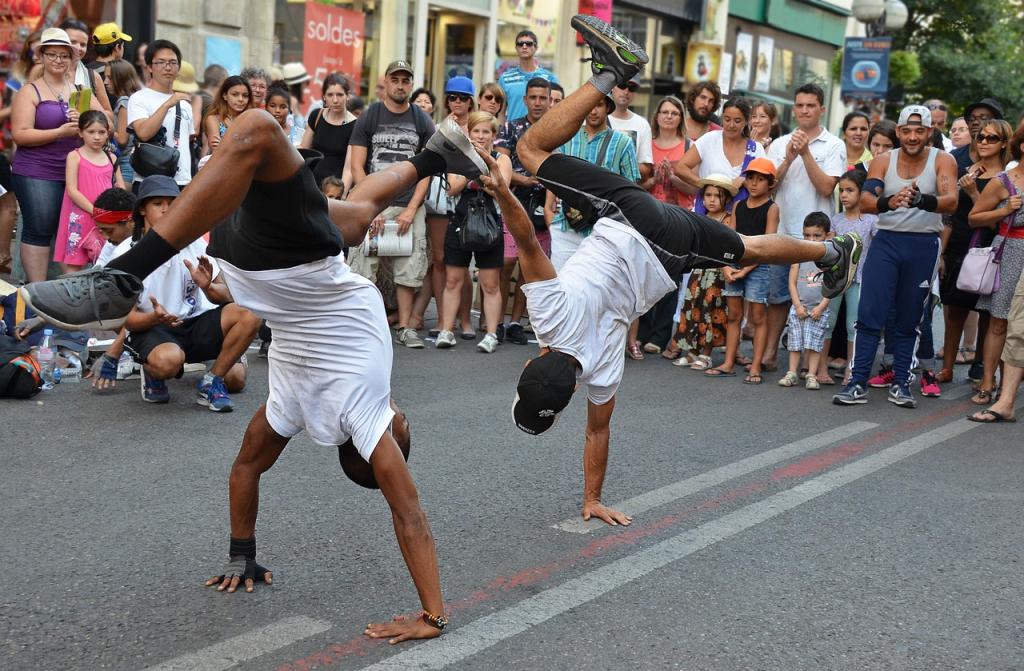In this vibrant street scene, two black men are captivating a crowd of onlookers with their impressive breakdancing skills. The performers are in the middle of a city street, marked with white dashed and solid lines, and flanked by small shops. The man on the left is upside down, balancing on both hands—one of which sports a weightlifting glove—while his legs kick out in opposite directions. He wears a white T-shirt, black shorts, and gray tennis shoes. Beside him, the second performer balances on one arm, his raised free arm stretching vertically. He too wears a black cap, white T-shirt, black shorts, and black tennis shoes, with both legs extending upward. A lively crowd, consisting of people of various ages but predominantly in their 20s and 30s, encircles them, watching with rapt attention. The bustling street backdrop, filled with vibrant colors—gray, white, red, black, brown, pink, purple, green, and blue—adds to the dynamic energy of this midday urban performance.